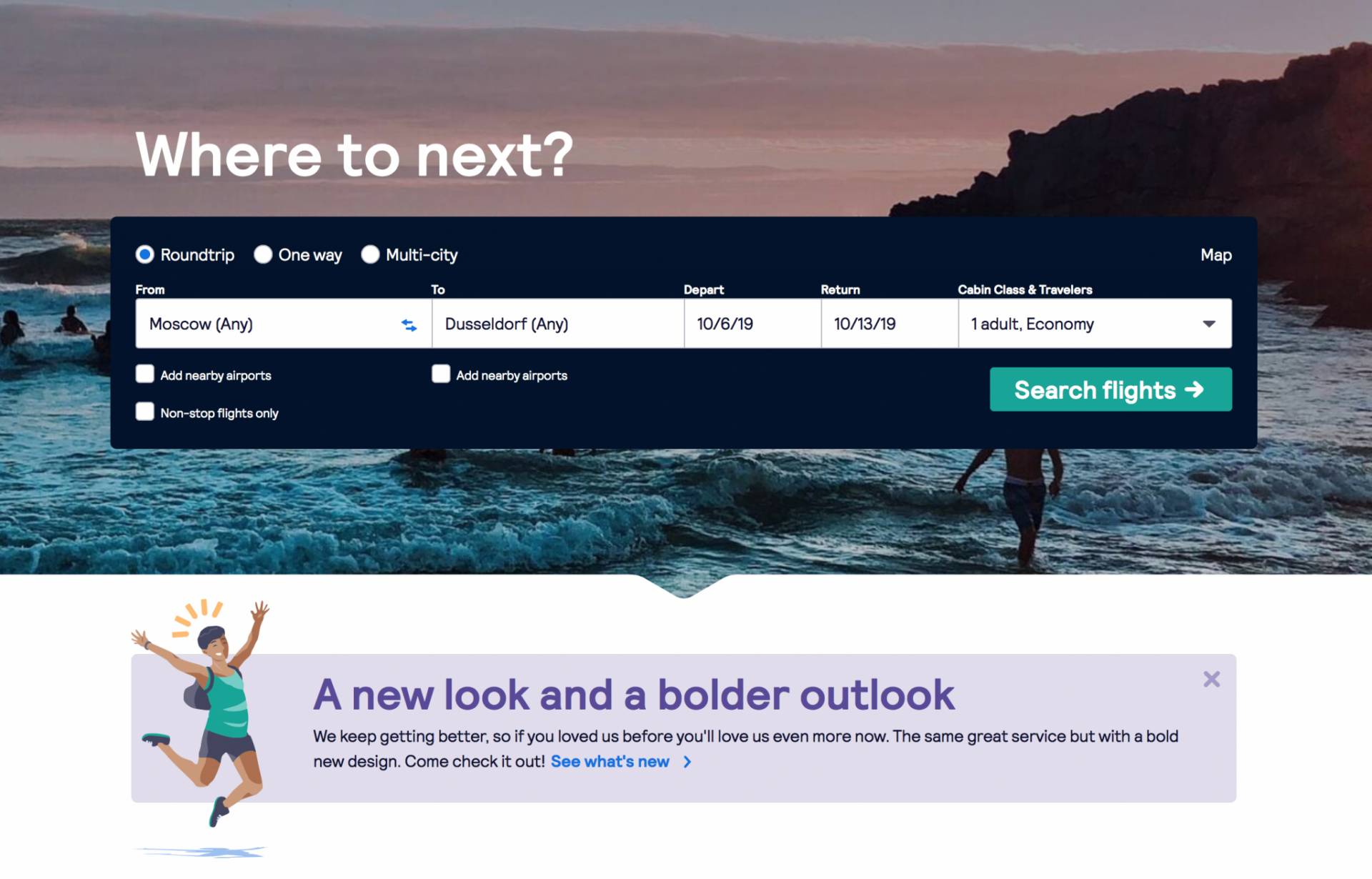**Detailed Caption:**

This image is a screenshot from a travel booking website. Dominating the visual is a hero image of a serene beachscape during the late evening or early morning. The beach features a group of people enjoying the water. In the background to the right, large rocks create a picturesque frame against the incoming waves. On the left, several people can be seen swimming in the foamy, dark grayish-blue ocean, illuminated by the fading light. The sky above transitions from a light blue at the top to a medium grayish-pink towards the horizon, suggesting the sun has either set or is obscured by a mountain range.

Central to the image is a wide blue rectangle spanning horizontally across the screen. This section contains the primary booking options. The search panel offers selections for 'Round Trip', 'One-Way', and 'Multi-City' flights. Currently, 'Round Trip' is selected. The departure city is listed as Moscow with the destination set to Dusseldorf. The travel dates indicate a departure on 10-16-19 and a return on 10-13-19. The selected travel preferences are for one adult flying in economy class. Additional options provided include adding nearby airports for both departure and return, and choosing non-stop flights only, though none of these are selected at the moment. A prominent teal button on the right of the blue panel is labeled 'Search Flights'.

Below the search options, a graphical banner showcases an adventurer jumping with a backpack, suggesting the exhilaration of travel. Accompanying the graphic is a promotional message: "A new look in Boulder Outlook. We keep getting better, so if you loved it before, you'll love us even more now. The same great service with the bold new design. Come check it out, see what's new." This encourages users to explore the newly enhanced features and design of the site.